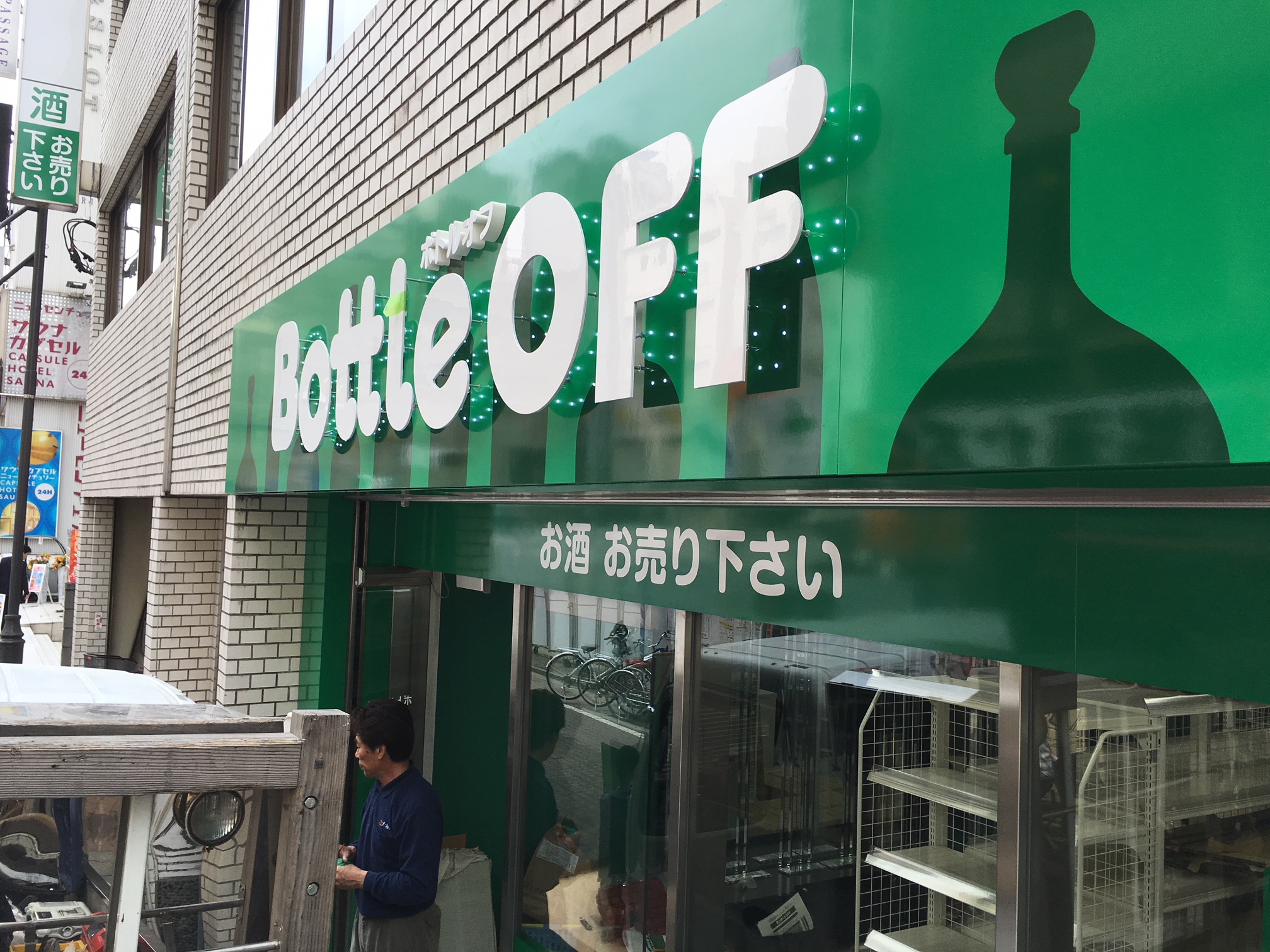The photograph captures an outdoor daytime scene of a storefront in an Asian city. The image is rectangular, approximately five inches tall and six inches wide, taken from a slightly elevated angle, about 30 degrees, looking down at the side of the building. 

The building, constructed with light gray-brown brickwork, is closer to the viewer on the right and extends further away to the left. Dominating the upper right corner is a green sign with large white letters that read "BOTTLE OFF," accompanied by a dark green image of a bottle top. Above this sign, there is a smaller green sign featuring white Japanese characters, which continue across a green banner centered over the shop's glass storefront windows.

The windows reveal empty racks inside the shop. In the lower left corner of the image, a man of Japanese descent, with black hair, light brown skin, and dressed in a long blue sleeve shirt and gray pants, stands facing left. A vehicle with wooden posts in its back is parked in front of the store. Further down the street, additional signage includes a blue or black sign pole with a white and green sign above it.

Overall, the storefront presents a clean and handsome appearance with its multi-storied structure, the second story featuring windows, and a small veranda-like structure extending from the building's facade.